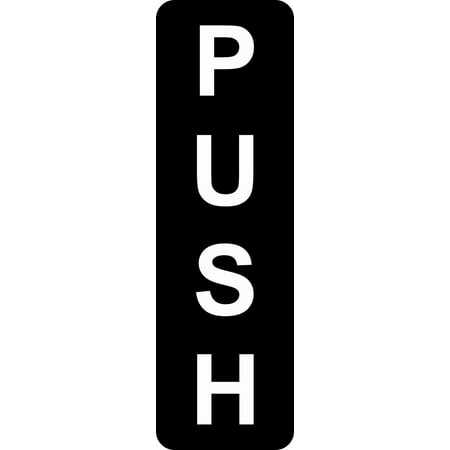The image features a vertical, black digital logo or sign positioned centrally against a completely white background. The design resembles a door sign or an instruction button, characterized by a long, black rectangle with rounded corners. Inside the rectangle, the word "PUSH" is displayed in bold, white letters, arranged vertically with one letter per line. The straightforward and legible font underscores the simplicity and clarity of the design, making it easy to read. The minimalist use of only black and white colors emphasizes the message, creating a stark yet functional visual.